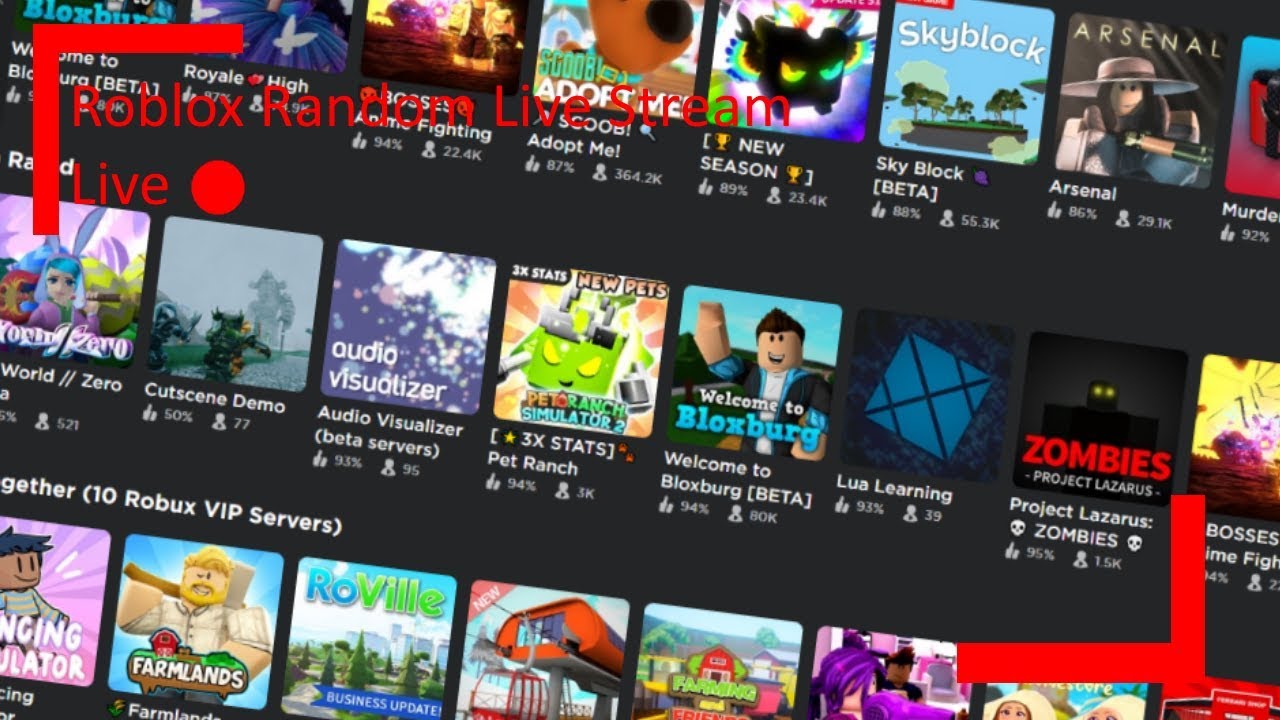The image depicts a promotional advertisement for Roblox, presented in a style reminiscent of Netflix's interface. It features a grid of various live streams, showcasing numerous creators actively playing Roblox. Each stream is represented by vibrant thumbnail images, similar to series posters, providing a visual preview of the content. For example, one thumbnail resembles a Scooby-Doo theme but focuses on a game called "Adopt Me," indicating its popularity with 875 participants and 364 viewers.

Underneath each thumbnail, detailed information is provided, including the title of the game or stream, player counts, and sometimes the number of current viewers, akin to subscription and view metrics on YouTube. The advertising layout organizes these streams into rows, with white text on a black background for descriptions, making them stand out against the colorful thumbnails. The headers and some elements like the "Roblox Random Live Stream" title are challenging to read due to their red font on a busy backdrop, which includes various design elements and pictures.

Additionally, the design incorporates minimalist red borders at the top left and bottom right corners of the interface, framing the content without enclosing it fully. This stylish touch, along with the comprehensive and interactive array of visual and textual information, aims to engage potential users by showcasing the immersive and diverse live stream offerings available on Roblox.